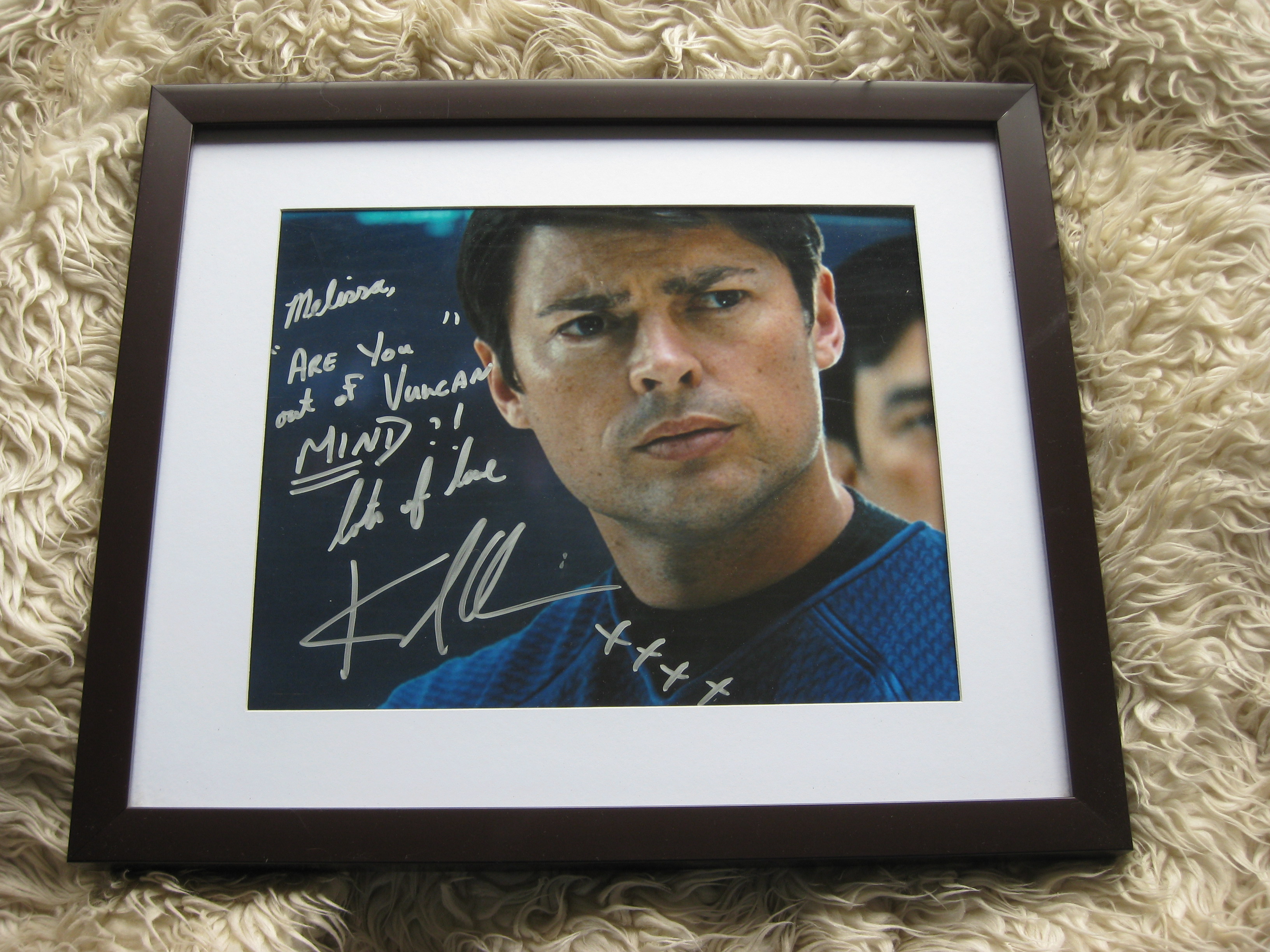The image depicts an autographed photo of a Hispanic actor in a dark brown frame, positioned on a shaggy carpet. The frame has a white matting that creates a border around the photo centered within it. The actor, with short, styled, combed-over hair, gazes off-camera with a neutral expression. He wears a light blue shirt featuring a pattern. An Asian gentleman stands slightly in front of him to his left, partially obscured. The autograph appears on the left side of the photo, with a legible phrase "Are you out of Vulcan mind?" followed by an indistinct cursive message. The autograph includes a series of "X"s extending over the actor's torso.